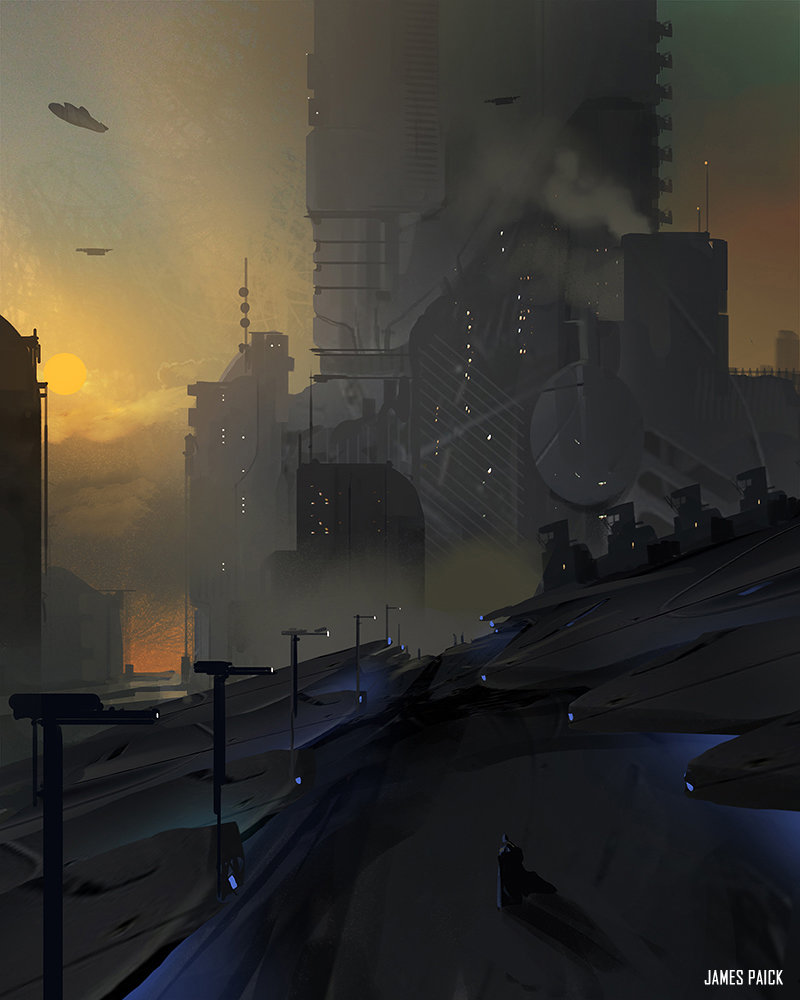This detailed digital artwork by James Paick features a striking futuristic cityscape dominated by a tall, central gray tower, partially obscured by the image's upper edge. Tiny specks of light, possibly window illuminations, punctuate its façade. The foreground reveals a large, tilted black street, lined with oddly shaped streetlights, adding to the scene's avant-garde ambiance. Notably, several oval-shaped aircraft hover near the tower, enhancing the futuristic feel.

In the background, a low-hanging sun, possibly setting, infuses the sky with a gradient of hazy oranges and yellows, deepening the dystopian tone. The skyline appears shrouded in smoke and haze, emanating from chimney-like structures on the building, contributing to the dramatic atmosphere. A pair of binoculars with white dots at the ends is noticeable in the foreground, though their purpose remains ambiguous.

The artist's signature, "James Paick," is subtly inscribed in white in the lower right corner, affirming the creation's identity and intricate detail.